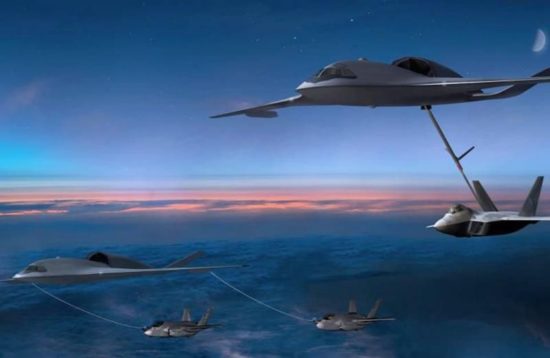In this striking aerial photograph, a deep blue sky transitions to a lighter blue at higher altitudes, with a captivating pink and orange sunrise hue gracing the horizon. The image, captured far above ground level, possibly over an ocean with some cloud coverage, showcases five sleek, military-style aircraft engaged in mid-air refueling maneuvers. Prominently featured, two primary aircraft each extend fuel hoses to smaller jet-like fighter aircraft. One primary aircraft, displaying a distinctive design with diagonally upward tail wings, uses a single fuel line to refuel a smaller jet beneath it. Simultaneously, another primary aircraft, characterized by an advanced, streamlined profile with a glass cockpit and a prominent engine housing, dispenses two fuel lines to refuel two fighter jets below. This scene exemplifies a high-altitude refueling operation with extraordinary visual clarity and depth.